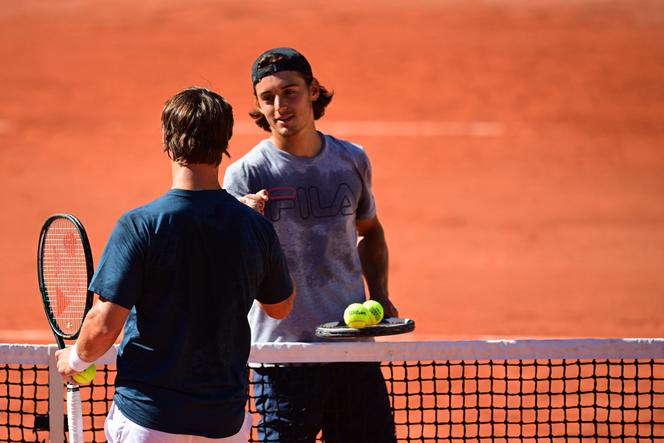The image captures a blurred rusty red background, possibly a wall or floor. In the foreground stands a tennis net, featuring a white top and black netting. Two men are positioned on either side of the net. The man on the left sports a dark blue shirt, white shorts, and has brown hair. The man on the right, also with brown hair, wears a backward black baseball cap, a gray shirt, and blue shorts. His appearance suggests he is very sweaty. Both men hold tennis rackets in their left hands; one racket is held vertically, while the other is horizontally balanced with two or three tennis balls resting on it. With their right hands, they engage in either a fist bump or handshake, likely marking the conclusion of their tennis match.